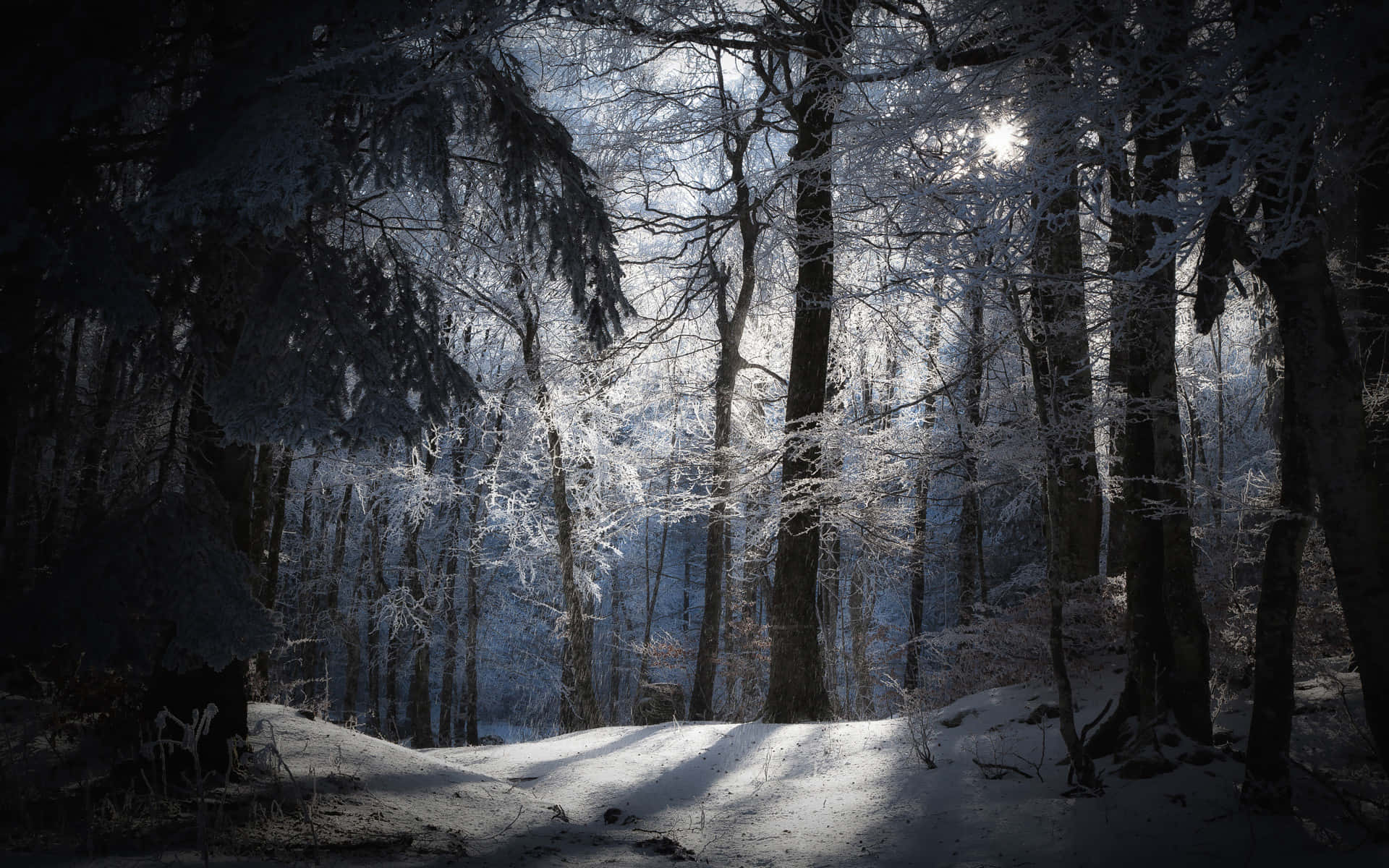Against a steel blue sky, the scene unfolds in a picturesque, snowy forest. The ground is blanketed in a gentle layer of snow, particularly illuminated in the bottom center by a mysterious white light that filters through the dense canopy. This light source emanates seemingly from the upper right corner of the image, casting a soft glow that contrasts sharply with the darker, shadowed areas on either side. Tall, dark trees stand in stark silhouette, their limbs intertwined and accented with patches of snow. The background is a tapestry of black tree branches and snowy accents, contributing to the ethereal quality of the forest. The overall image is crisp and vivid, capturing the quiet, serene beauty of the natural scene, devoid of any signs of human or animal presence.